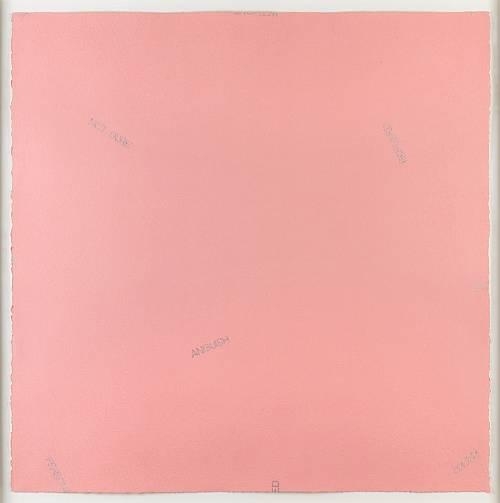The image depicts an abstract, computer-generated piece of art predominantly featuring the color pink. Set within this pink square are scattered, light gray letters that spell out the word "Ambush" multiple times. The pink background, described as a muted salmon color, nearly fills the entire square, leaving a small, even white border on all four sides. This border is a cloudy bone white, contrasting subtly with the pink. The pink area shows some irregularities, where the left and right edges appear torn and jagged while the top and bottom edges are more cleanly cut. Within the pink square, the word "Ambush" repeats five times in light gray text, blending subtly with the background, making it hard to read. The letters overlap and are distributed across various parts of the image, contributing to its abstract nature. There are also some additional, undecipherable markings or possible letter combinations like "N-C-7" sporadically placed around the square. This artwork, possibly a painting or photograph, gives a modern, minimalist impression with its simple yet complex layering of text and color.